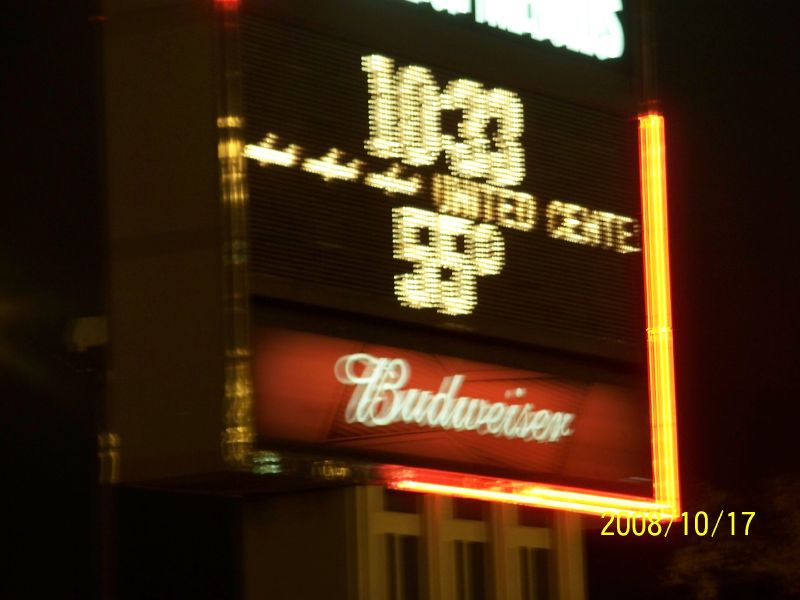This square color snapshot captures a neon sign at night, with a timestamp in the lower right-hand corner reading "2008/10/17". The sign is slightly blurred against a completely dark background, save for a few windows visible below the sign. The top part of the sign features very bright, yet illegible, white neon letters. Below, there's a digital clock displaying the time as 10:33. Further down, it states "United Center" along with an indication of the temperature, "55 degrees", both illuminated in lights. Additionally, the middle section includes three airplane illustrations done in lights. The bottom of the sign features a red strip with a white cursive advertisement for Budweiser beer. Surrounding the entire sign is yellow neon, highlighting its edges.